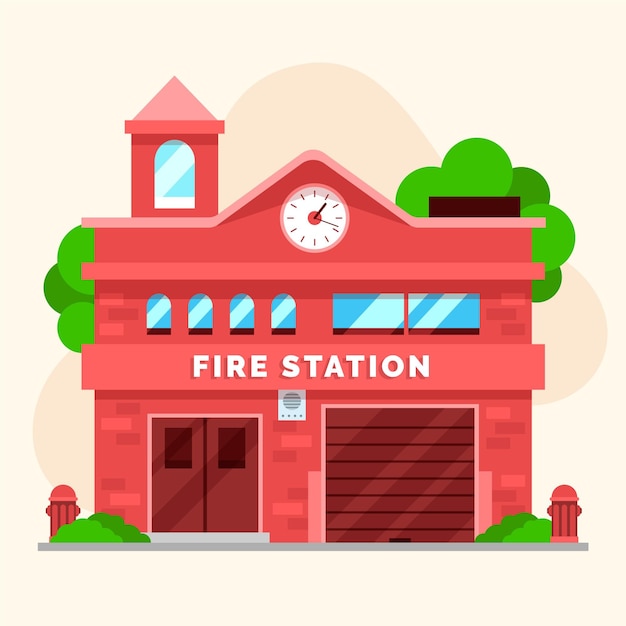This illustrated image of a fire station depicts a cartoon-esque scene bursting with vibrant, colorful details. Dominated by a cheerful bright red hue, the fire station features a prominent white sign across the top that reads "Fire Station." Below the sign is the large red garage door, distinctively darker than the rest of the building, where fire trucks would be housed. Adjacent to the garage door are two double doors, providing additional access to the station.

A small speaker is positioned beneath the "Fire Station" sign, adding to the station's functional details. Above the sign, two rectangular windows are set side-by-side, directly over the garage door. The other side of the building showcases four arch-shaped windows, contributing to the structure's architectural charm.

Crowning the building is a clock, perched high above, and a petite tower with a single window, enhancing the classic fire station silhouette. The left-hand side of the image reveals some trees peeking from behind the station, indicating the presence of a nearby park or wooded area. Adding to the scene’s realism, two shrub bushes adorn each end of the building, while two bright fire hydrants stand ready at their posts—one to the left and the other to the right of the station. This richly detailed image encapsulates the iconic and bustling aesthetic of a quintessential fire station.